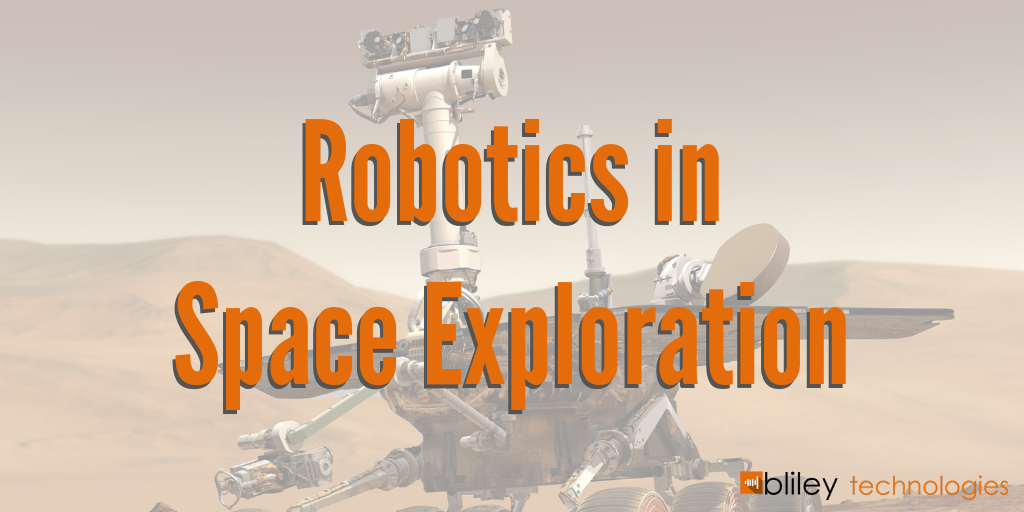This image appears to be a banner or advertisement in a horizontal rectangular format. Dominating the center, slightly above the middle, is bold orange text with a solid dark gray drop shadow, reading "Robotics in Space Exploration." The first letters of "Robotics," "Space," and "Exploration" are capitalized, while "in" is in lowercase. The background image is somewhat hazy and with reduced opacity, featuring a robotic rover reminiscent of those used for Mars exploration. This rover includes intricate details like rods extending to the surface, wheels at the bottom, and a small white tower at the top with sensors and cameras. The backdrop displays a light gray sky and a sandy brown desert-like landscape with distant hills. In the bottom right-hand corner, a logo is present, with "BILLEY" spelled out in black letters, followed by "Technologies" in smaller orange text.